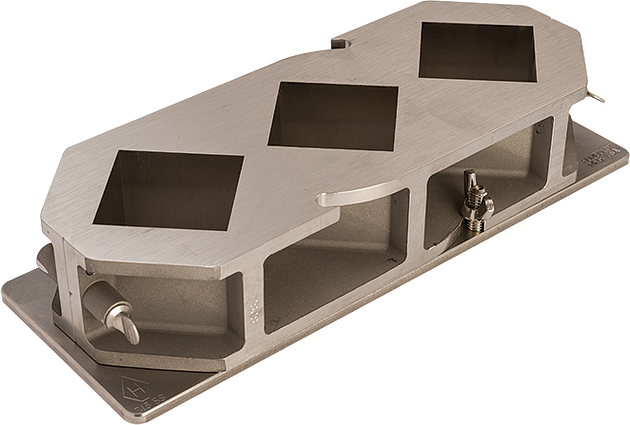This image depicts a molded plastic piece of equipment without a border, comprising three pieces—a top section, a bottom section, and a middle part potentially accessed by separating the structure. The top section features three evenly spaced, diamond-shaped square cutouts that penetrate through the material, possibly for functional purposes or as part of its design. The overall object gives the impression of a molding block, with the top piece consisting of two interconnected parts, both affixed to a bottom rectangular plate with screws or bolts. A twisty nut and another bolt on the bottom right are visible, suggesting the mechanism can be disassembled. Additional details include engraved markings, such as an 'H' and the identifier 'B1853,' further hinting at the equipment’s industrial or specialized nature. The background of the image is white, implying it was photographed on a flat surface for clarity.